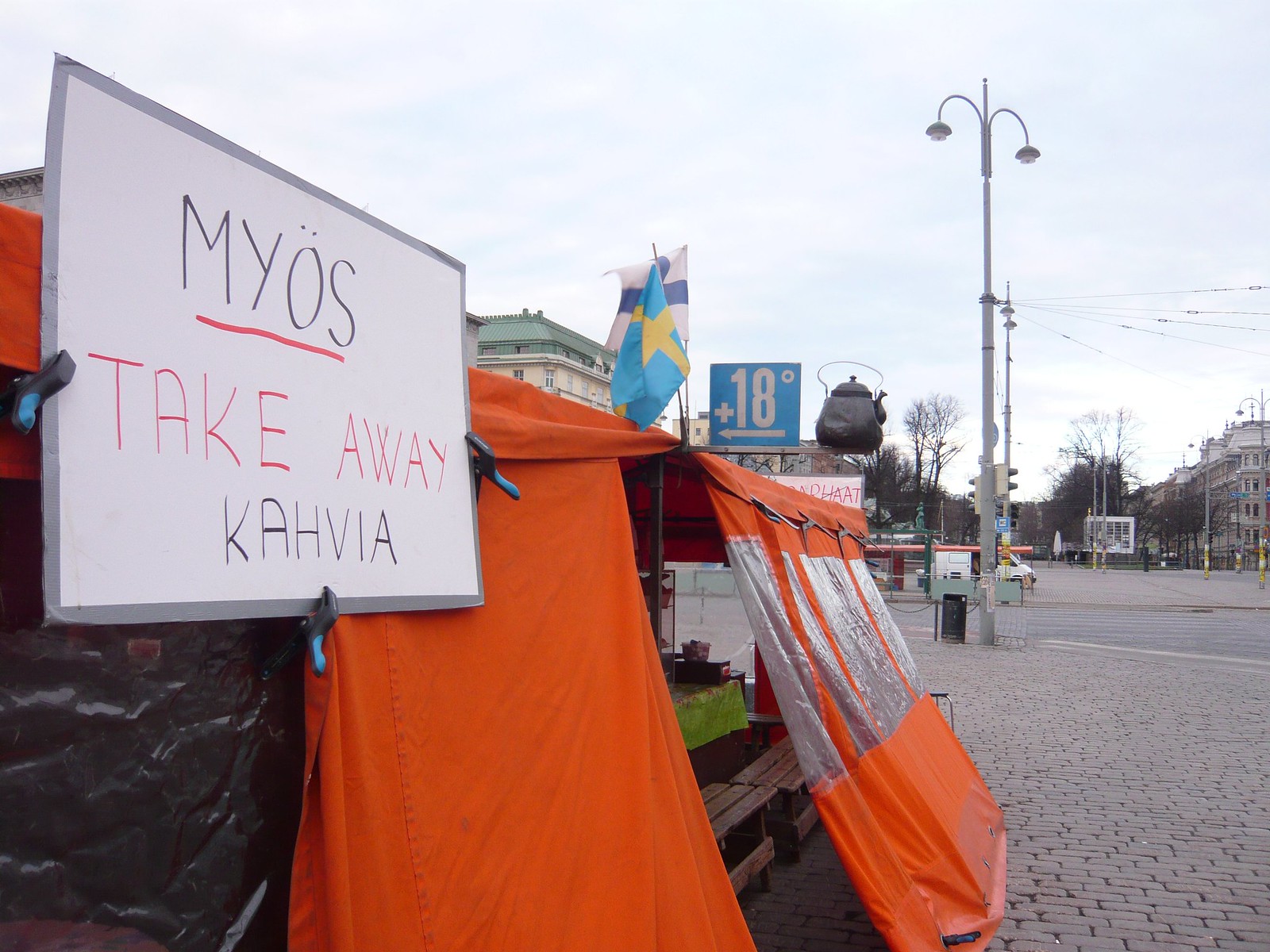The image depicts a bustling street scene with cobblestone pavement, likely in a modern area with old-world charm. Various buildings, some tan with gray roofs and others yellow with green roofs, frame the sides of the street. In the center foreground, an eatery with an orange canopy and sides immediately draws attention. Inside the canopy, wooden tables and benches are set with green tablecloths and various items. At the entrance, a handwritten sign on a whiteboard stands out. The sign, featuring black and red letters, prominently displays "MYOS" underlined in red, followed by "TAKE AWAY" in red, and "KAVIA" in black. The weather is gloomy, with overcast skies casting a grayish tint over the scene.

Additional details enhance the locale's character: a streetlight and a tea kettle, possibly bronze, are seen hoisted up, adding a quaint touch. A nearby blue sign with white letters indicates "18+" with an arrow pointing to the left. The street and surrounding pavement are gray, contributing to the muted color palette, while the eatery contrasts with its vibrant orange canopy. Trees with mostly brown trunks and some sparse green leaves add a natural element. Overall, the scene merges historical architecture with modern amenities, creating a visually intriguing and atmospheric snapshot.